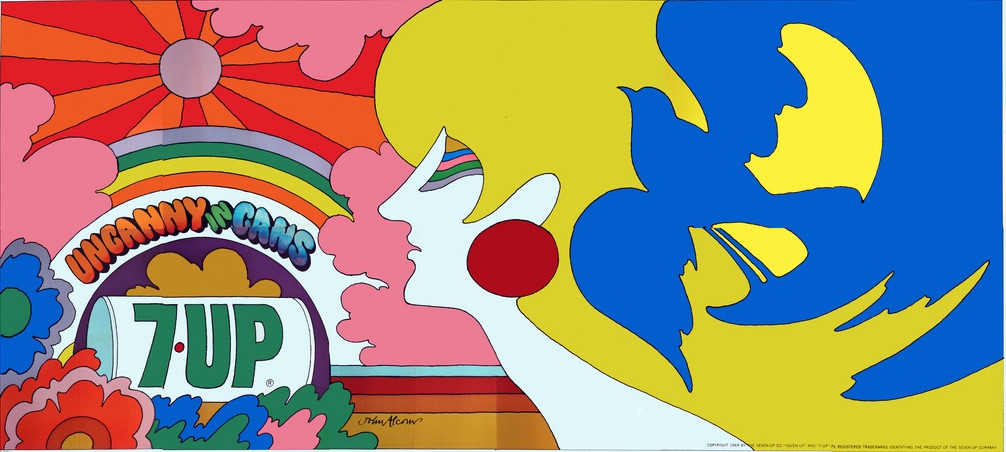This vibrant, retro-style artwork resembles a trippy 1960s advertisement. Dominated by a swirl of psychedelic colors—royal blue, banana yellow, bright red, forest green, pink, oranges, and purples—the image reveals intricate details that become apparent upon closer inspection. On the right, a bright blue form takes the shape of a bird, blending seamlessly into the yellow, which conjoins to create the hair of a stylized human silhouette. The face, outlined in white, features a multicolored eye with hues of brown, blue, green, and light purple arranged in a triangular shape, while a large red circle mimics an earring. Above, a light purple sun with red and orange rays illuminates the scene, surrounded by three pink clouds. Below the sun, a rainbow arches in shades of light purple, green, yellow, and orange, with the word "uncanny" in orange bubble letters. This is followed by "in" in green and "cans" in blue, forming the phrase "uncanny in cans." Beneath, a sideways white soda can displays the phrase "7 up" in sage green, with a red dot separating the number from the word. The composition concludes with several blue and orange flowers and green foliage, amplifying the image's vibrant, free-spirited essence evocative of classic hippie culture.